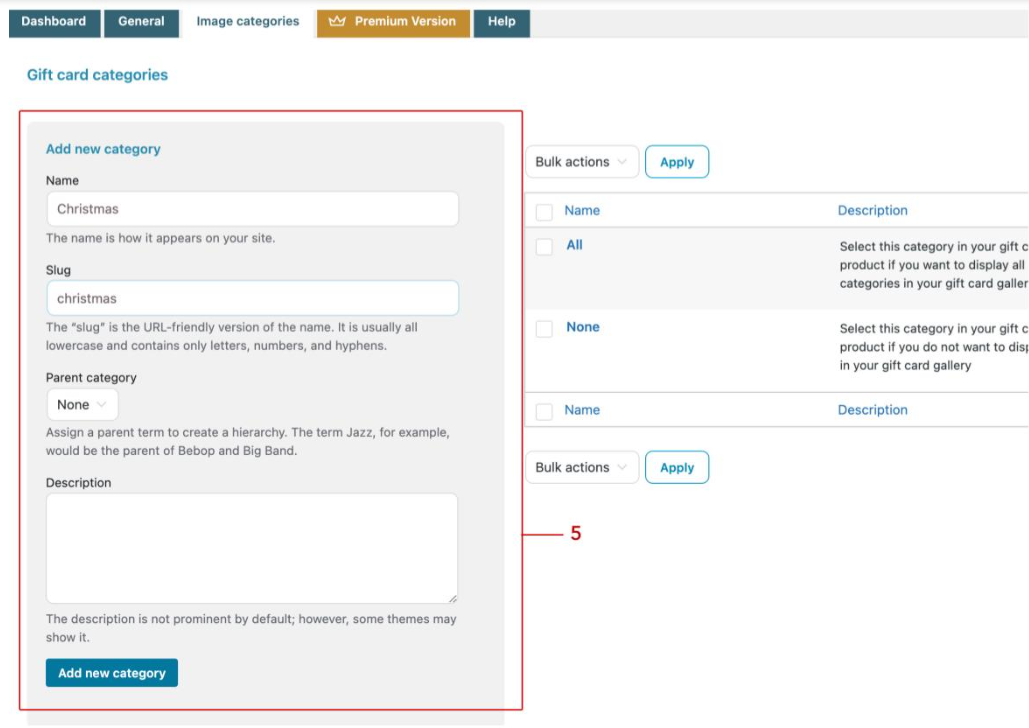The website displays a navigational menu at the top featuring tabs labeled "Dashboard General," "Image Categories," "Premium Version," and "Help." Except for "Image Categories," which is highlighted with a white background and blue text, the other tabs are blue with white lettering. The "Premium Version" tab also includes a gold crown icon.

Below the tabs, the main content of the page focuses on "Gift Card Categories," with a prominently highlighted box outlined in red. To the side of this, there's an illustration of a hand with five fingers extended. The box contains a blue-labeled "Annual Category" section with a currently selected category name, "Christmas," which indicates how it will appear on the site.

Further down, under the label, there's a slug input field pre-filled with "christmas," accompanied by a note that explains: "The slug is a URL-friendly version of the name, usually all lowercase and containing only letters, numbers, and hyphens." Below this is a "Parent Category" dropdown menu, currently set to "None," with a tooltip explaining that assigning a parent term helps create a hierarchical structure (e.g., "Jazz" could be the parent of "Bebop" and "Big Band").

There's also an empty "Description" text box labeled with information that a description is not prominently displayed by default but may be shown by some themes or plugins. At the bottom of this section, there's a blue "Add New Category" button.

To the right, there is another section for bulk actions, including a dropdown box labeled "Bulk Actions" and a button to apply the selected action. Below, there is a table with columns for "Name," "Category," and "Description," all of which currently contain no entries.